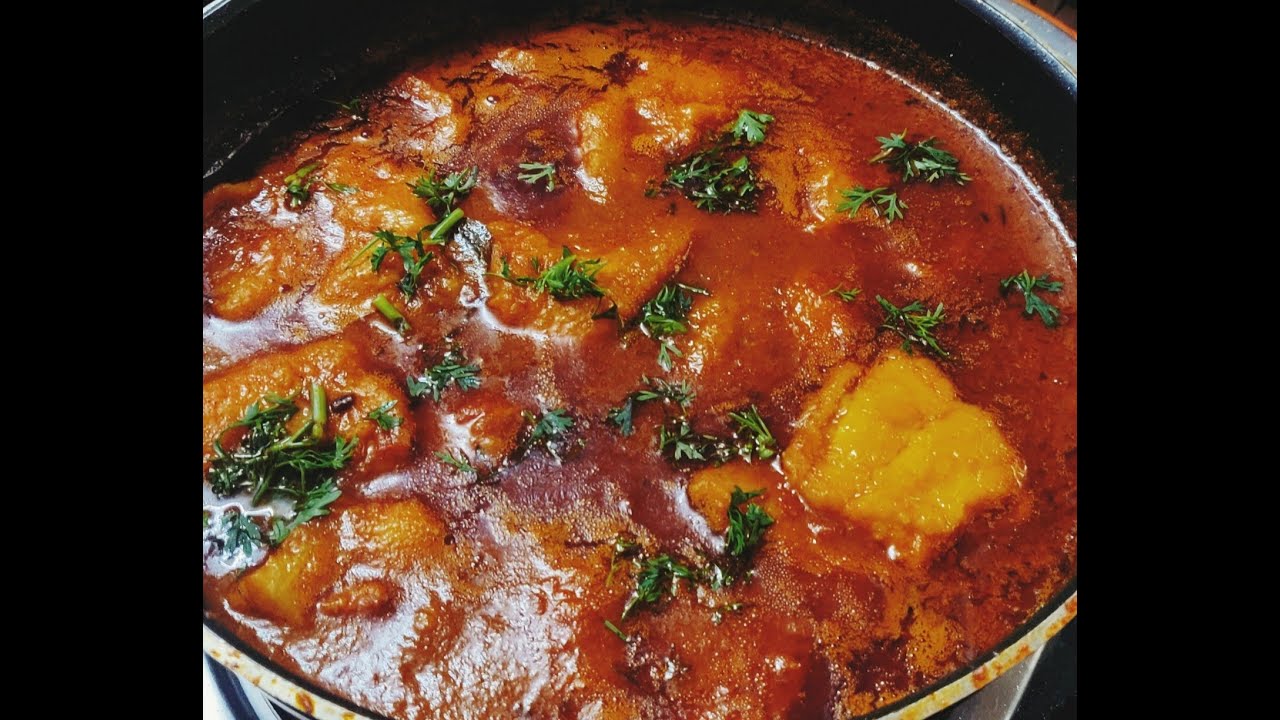This color photograph captures an overhead shot of a savory stew simmering in a silver metal pot with a black glazed interior, speckled with white spots. The stew itself is predominantly red, suggesting a tomato-based broth with a rich, bright hue. Floating atop are chunks of yellowish substance, possibly squash or a light-colored protein like chicken or fish, hinting at a dish similar to shakshuka or a red curry. The surface glistens with darker red fat and reflective white sections. Scattered abundantly across the top are fresh green herbs, akin to oregano or parsley, their stalks and leaves clearly visible. The background is black, with two black bands framing either side of the image, emphasizing the vibrant colors of the hearty, tomato-rich stew.